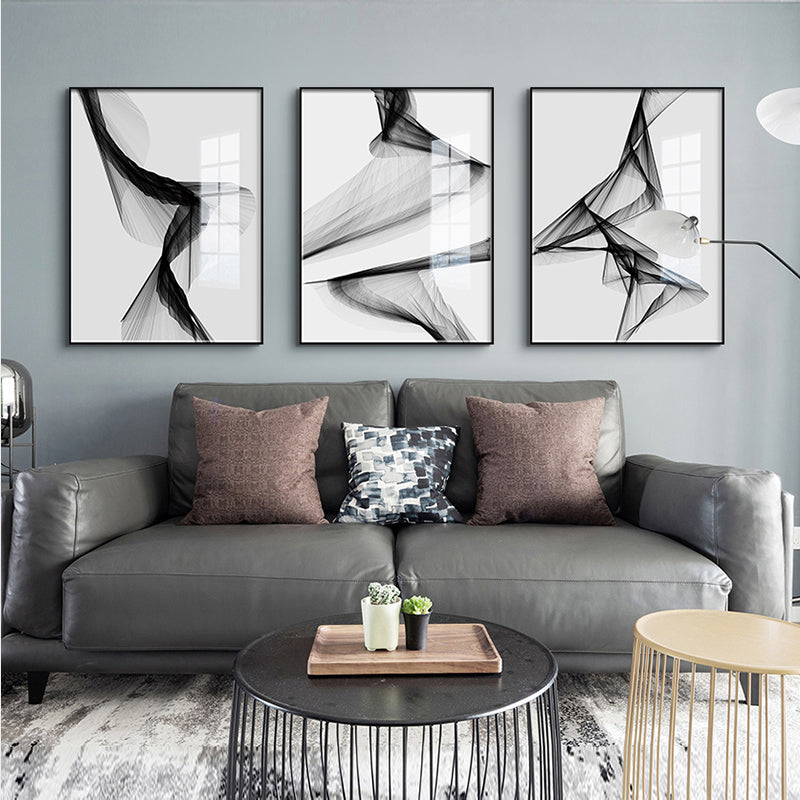The image showcases a beautifully decorated, magazine-worthy modern living room. The backdrop is a light smokish gray wall adorned with a unique triptych of abstract black and white artwork, each piece encased in a sleek glass frame that reflects nearby windows. This trio of images combines to form a cohesive geometric design on white backgrounds. Centered against this artistic backdrop is a plush, puffy gray couch, large enough for two, adorned with two reddish-brown pillows on the sides and a prominent white and blue pillow in the middle. The floor features a stylish black, white, and gray rug, contributing to the monochromatic theme, and underpins a round black coffee table. On this table rests a wooden tray holding two plants, a green leafy plant in a black pot, and a small dark green cactus, adding a touch of nature to the sophisticated space. Adjacent to the main coffee table is a smaller, very light brown wooden table, completing the elegant yet modern look of the living room.